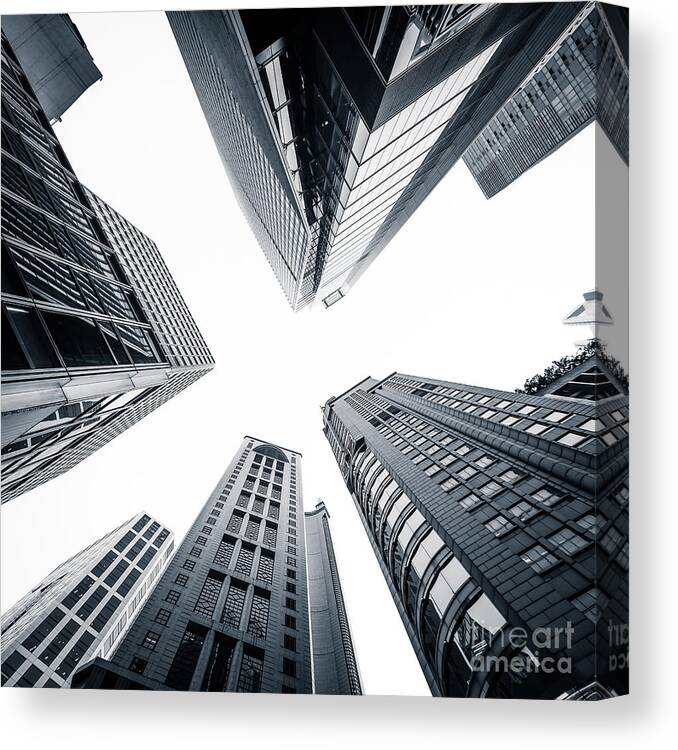The photograph is a striking vertical shot of four skyscrapers, taken from the ground, looking straight up to the sky, giving a sense of standing at the center of an urban canyon. These tall buildings, composed of dark concrete, steel, and glass, jut out from all angles, creating a striking contrast against the featureless, white sky. The high-contrast imagery gives the photograph an almost black-and-white appearance, despite it not being entirely monochromatic. The image is square and extends around the edges for a 3D effect, eliminating the need for a traditional frame. Notably, "Fine Art America" is inscribed in white lettering at the lower right corner, adding a subtle watermark to this cold, lifeless cityscape.